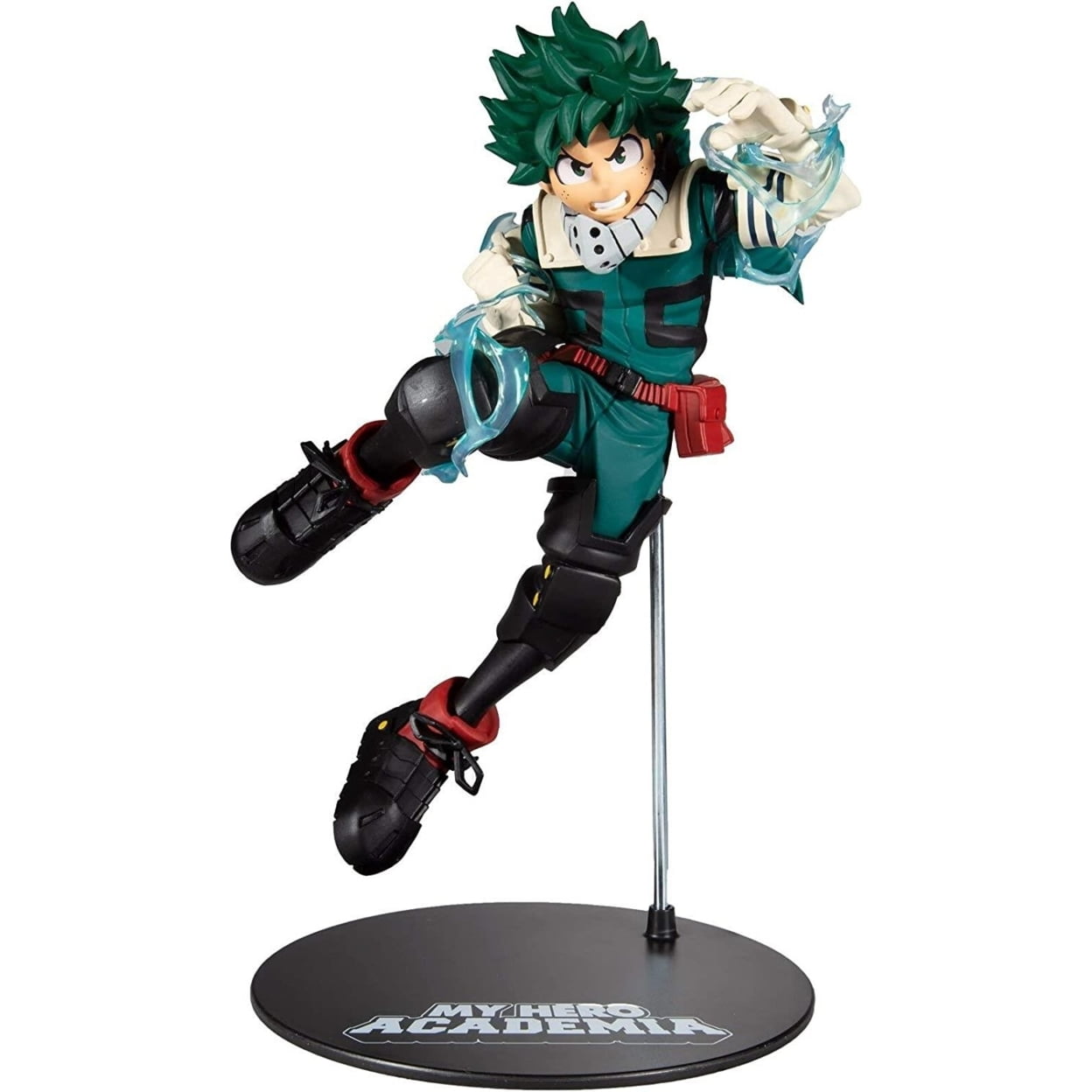The image depicts a high-quality, detailed figurine of Deku from the TV show "My Hero Academia," positioned against a plain white background. The figurine stands on a flat, round black base with the title "MY HERO ACADEMIA" printed in white capital letters. From the base, a thin metal rod ascends, supporting the character mid-air, giving the impression of jumping. Deku has distinctive green spiky hair and fair skin, with green, intense eyes framed by downward-slanted eyebrows, adding a fierce expression to his face. His teeth are gritted in a look of determination. He is dressed in a green bodysuit adorned with black knee pads, and a gray neck regulator or gas mask. He also wears white gloves, a red belt with a utility case, and black shoes highlighted with a red border at the ankles. Additional features include streams of water emerging from his hands, enhancing the dynamic and animated appearance of the figurine. The overall image is brightly lit, enhancing the clarity and colorful details of the figurine.